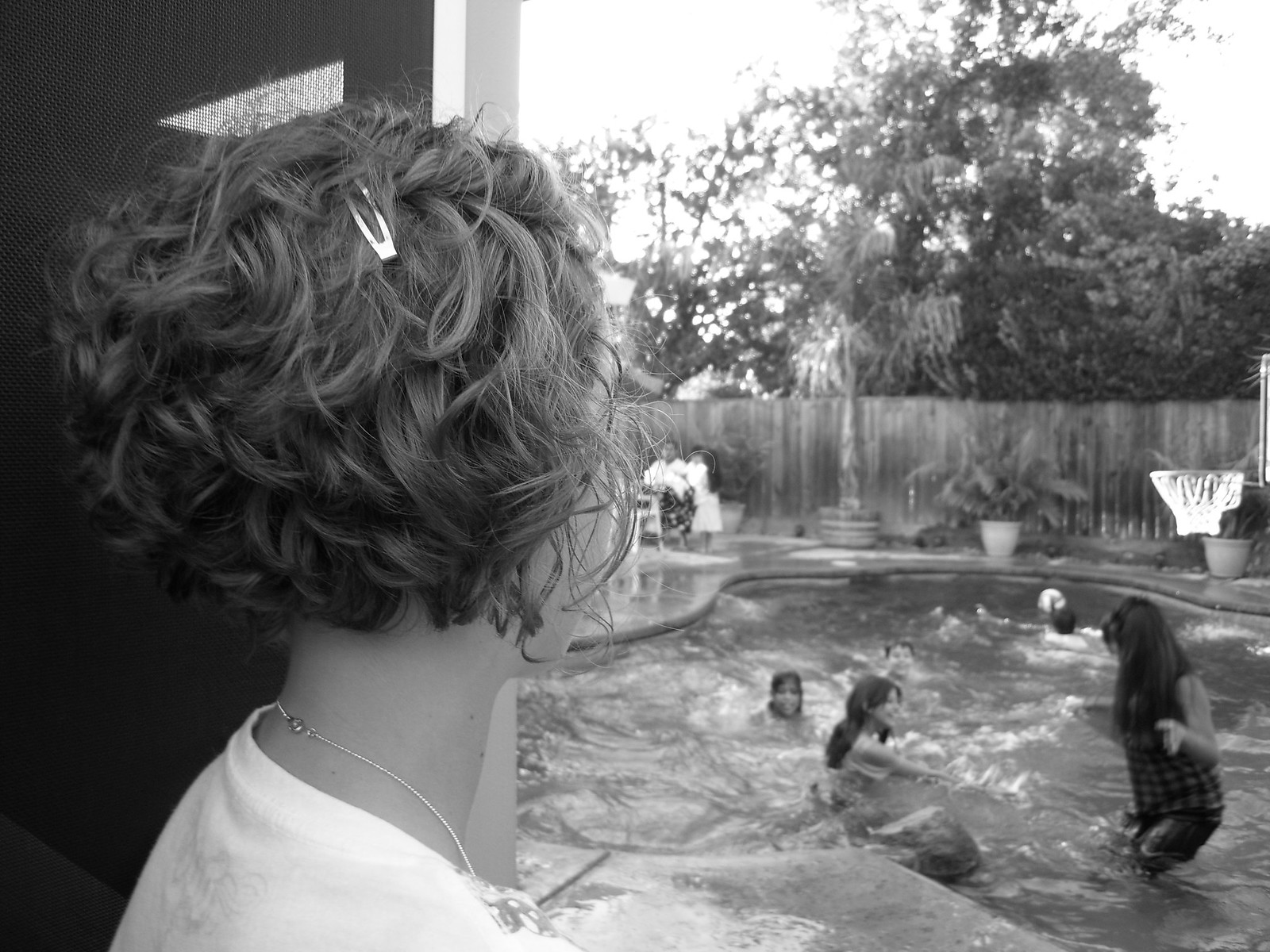In this black-and-white photograph, the left half of the image is dominated by a woman facing away from the camera. She has short, possibly brown, curly hair adorned with a silver barrette, and she appears to be Caucasian with paler skin. She is wearing a white shirt and a thin silver necklace with a visible clasp at the back. The right half of the image features a backyard pool with an irregular "amorphous blob" or oval shape, filled high with water. There are about four or five children of varying ages playing in the pool, some immersed up to their necks while one child near the far right edge stands slightly out of the water. The pool's stone deck is wet, and a basketball hoop is visible on the far right edge. In the background, a tall wooden plank fence with vertical boards separates the yard from a dense area of trees. The sky above is bright, almost white, casting a morning light that enhances the contrast of the scene. Details in the sky are lost due to the brightness.